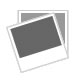The image prominently features a large, yellow McDonald's logo with the characteristic golden arches, made of a plasticky material, at the center. The logo is surrounded by a light blue outline against a white background, with some subtle shading. To the top left of the McDonald's M, there's a white road sign displaying "Route 66" in black lettering. Below the Route 66 sign, a wide red arrow points left, aligning with the same direction. The overall arrangement suggests a clip art style, potentially used for an advertisement, product example, or magnet, hinting at a location relation between McDonald's and Route 66.